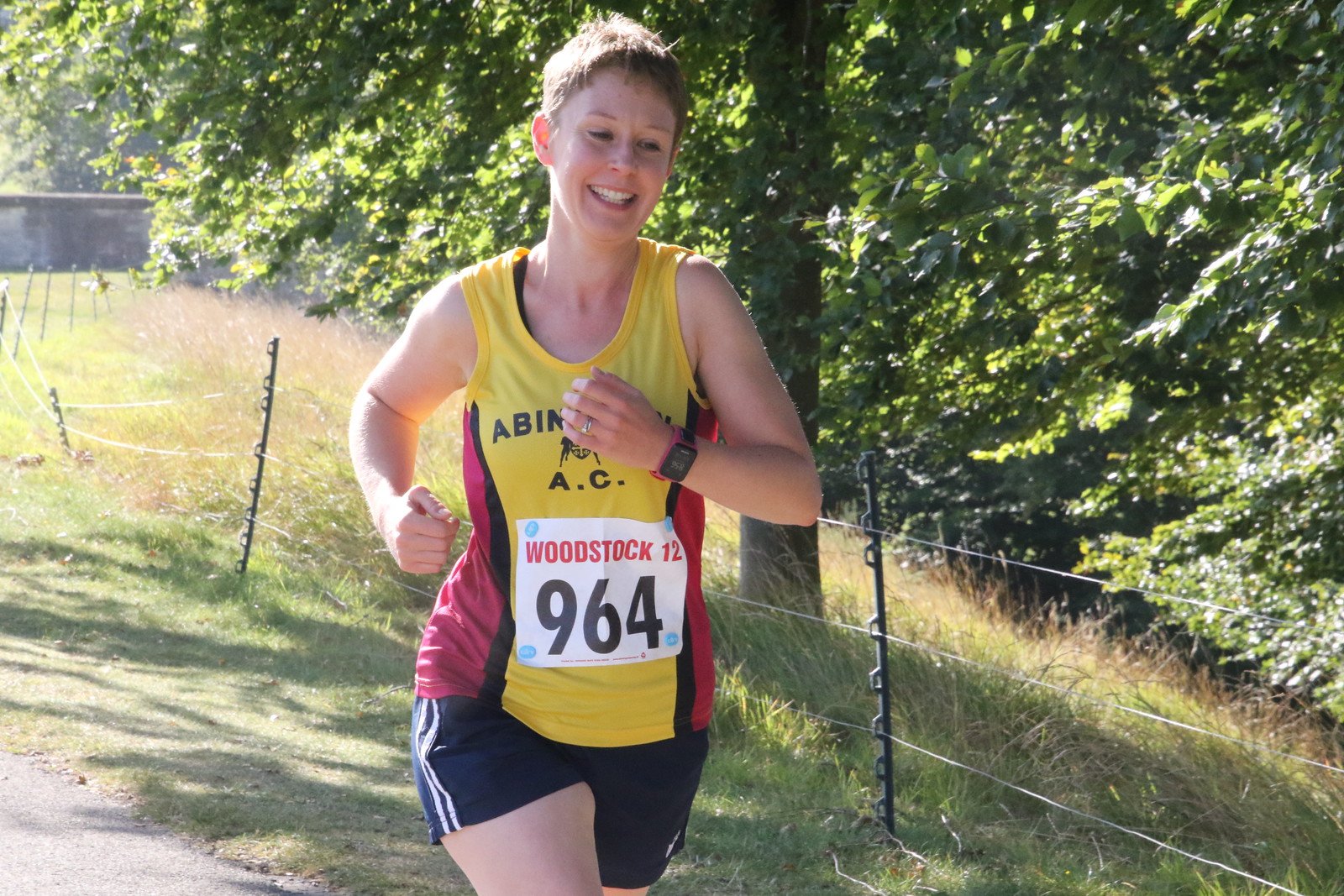This image captures a dynamic moment of a woman running in a race, likely a marathon, set outdoors along a road lined with grass and trees. The path is demarcated by strings held up by rods, forming a barrier. The runner, who is white with short blonde hair, dons a vibrant uniform: a yellow tank top with red and black accents, and black shorts with white stripes on the right side. Pinned to her chest is a race bib reading "Woodstock" with the number 964. She is smiling, appearing focused and joyful, with a red and black watch on her left wrist and a wedding ring on her hand. In the background, there are bushes, a prominent tree, and a distant wall, all contributing to the serene yet competitive atmosphere of the scene. The grass on the roadside is lush, contrasting with the road's paved surface, creating a vivid setting for her athletic endeavor.